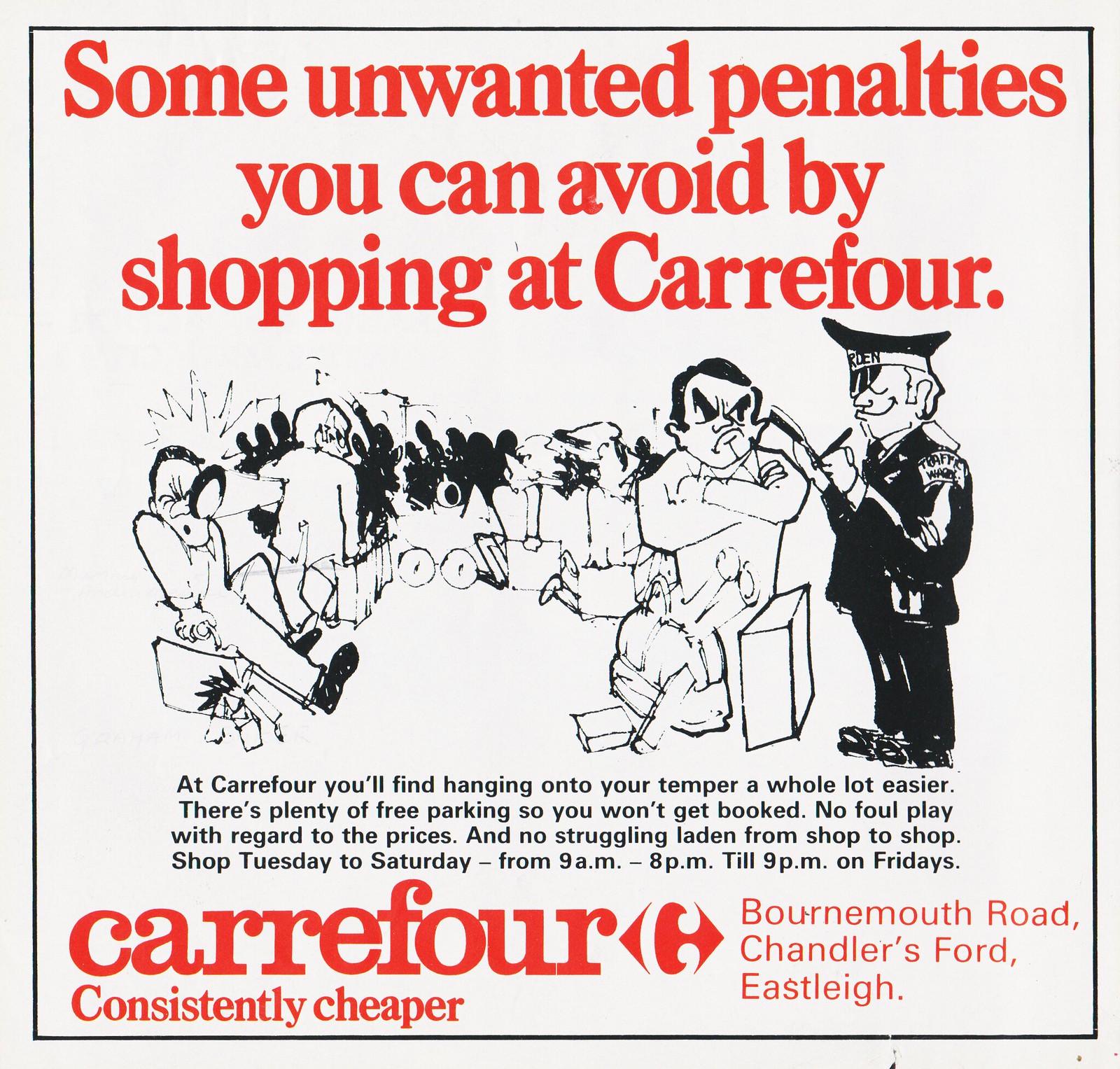This square advertisement for Carrefour Grocery is displayed on an aged white background, with prominent bright red text. At the top, in large font, it reads "Some unwanted penalties you can avoid by shopping at Carrefour." The central image is a chaotic black and white cartoon, capturing disgruntled shoppers and a police officer writing a citation. One man, angrily receiving the ticket, contrasts with the officer's smile. Meanwhile, another man carrying a briefcase and a log is hit, adding to the scene’s mayhem. Below this, there is small black text stating, "At Carrefour, you'll find hanging on to your temper a whole lot easier. There's plenty of free parking so you won't get booked. No foul play with regard to the prices and no struggling laden from shop to shop. Shop Tuesday to Saturday from 9 a.m. to 8 p.m., till 9 p.m. on Fridays." At the bottom, in bold red lowercase letters, it asserts, "Carrefour, consistently cheaper." The location is provided as Bournemouth Road and Chandler's Ford in Eastleigh.